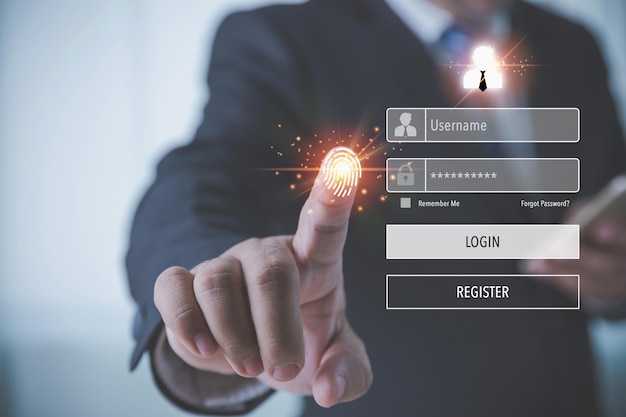The image is a rectangular login screen, wider than it is tall, featuring a blurry background of a man in a business suit. The man, dressed in a dark suit with a white shirt and a slightly faded blue tie, is holding a phone in his left hand. His right hand is extended towards the screen, with his pointer finger touching it, creating the appearance of a bright yellow and orange glowing fingerprint. Sparkles and orange specks radiate from his fingertip.

In the foreground, the login interface is displayed prominently. To the right of the glowing fingerprint, there is a gray box labeled "username" accompanied by a silhouette of a man in a suit. Below it, a "password" box features a padlock icon and a row of 10 asterisks. Additionally, there is a checkbox labeled "remember me" with a "forgot password" option next to it. At the bottom of the screen, there are buttons labeled "login" and "register". The overall setting has a white, somewhat bright background, indicating a modern, tech-focused theme.